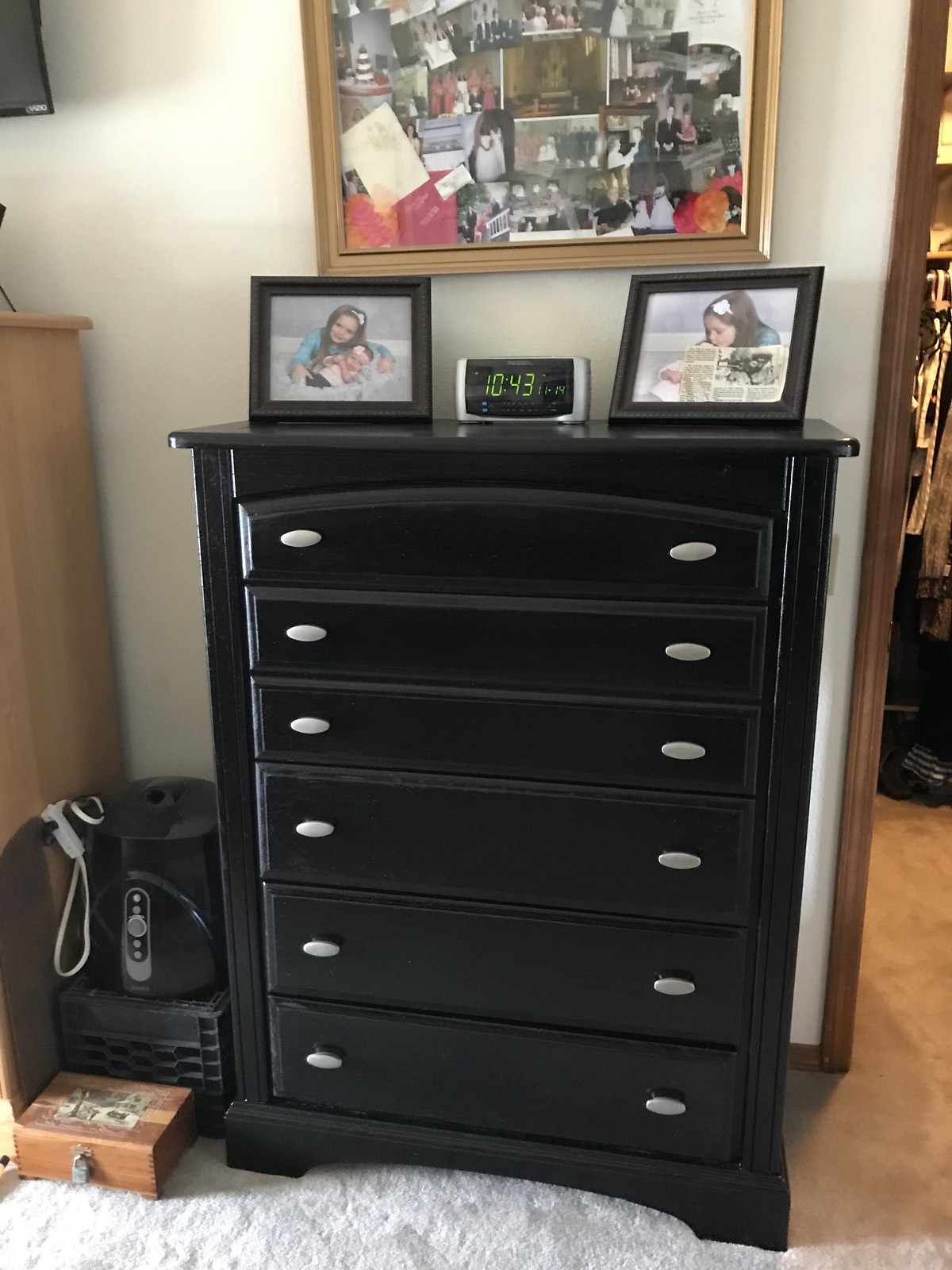This photograph captures a section of a bedroom, prominently featuring a tall, black wooden chest of drawers with six drawers, each adorned with two oval-shaped silver handles. Sitting atop the dresser are two black-framed photos, both depicting a young girl with a baby, though one of them is partially obscured by a newspaper clipping. In between the photographs is a silver digital alarm clock showing the time as 10:43 in green digits against a black face. Above the dresser hangs a large gold-framed collage displaying an assortment of smaller family photographs. To the left of the dresser, on the floor, is a small wooden box with a lock, topped by a black crate, and what appears to be a black air fryer. Partially visible on the left side of the image is a light brown dresser and a possible TV mounted on the beige wall. To the right of the black chest of drawers, there's an open doorway leading to a closet, where clothes are hanging and items are strewn on the tan carpet. The main room's carpet is light gray.